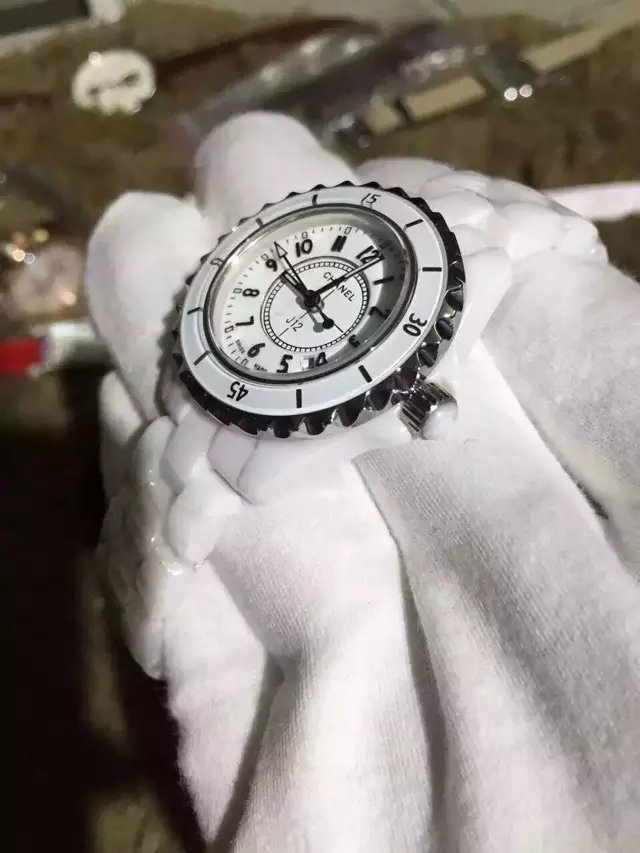This captivating photograph showcases a luxurious Chanel J12 analog wristwatch, exuding elegance and sophistication. The timepiece features a stunning white-on-white color scheme, which enhances its refined aesthetic. The interior dial is emblazoned with "J12" and marked with luminous hour, minute, and second hands that glow in the dark. The circular dial is meticulously detailed, with clear analog numbers adding to its classic appeal.

The outer bezel, made from highly polished silver stainless steel, includes adjustable indicators at 15, 30, 45, and 0 minutes, providing functionality and style. The adjustment knob mirrors this high-end design, crafted from what appears to be ivory, adding a touch of opulence. The strap seamlessly continues this luxurious theme with an ivory-like appearance, completing the watch's exquisite look. This Chanel J12 analog watch encapsulates an unparalleled sense of luxury and craftsmanship, making it an undeniable statement piece.